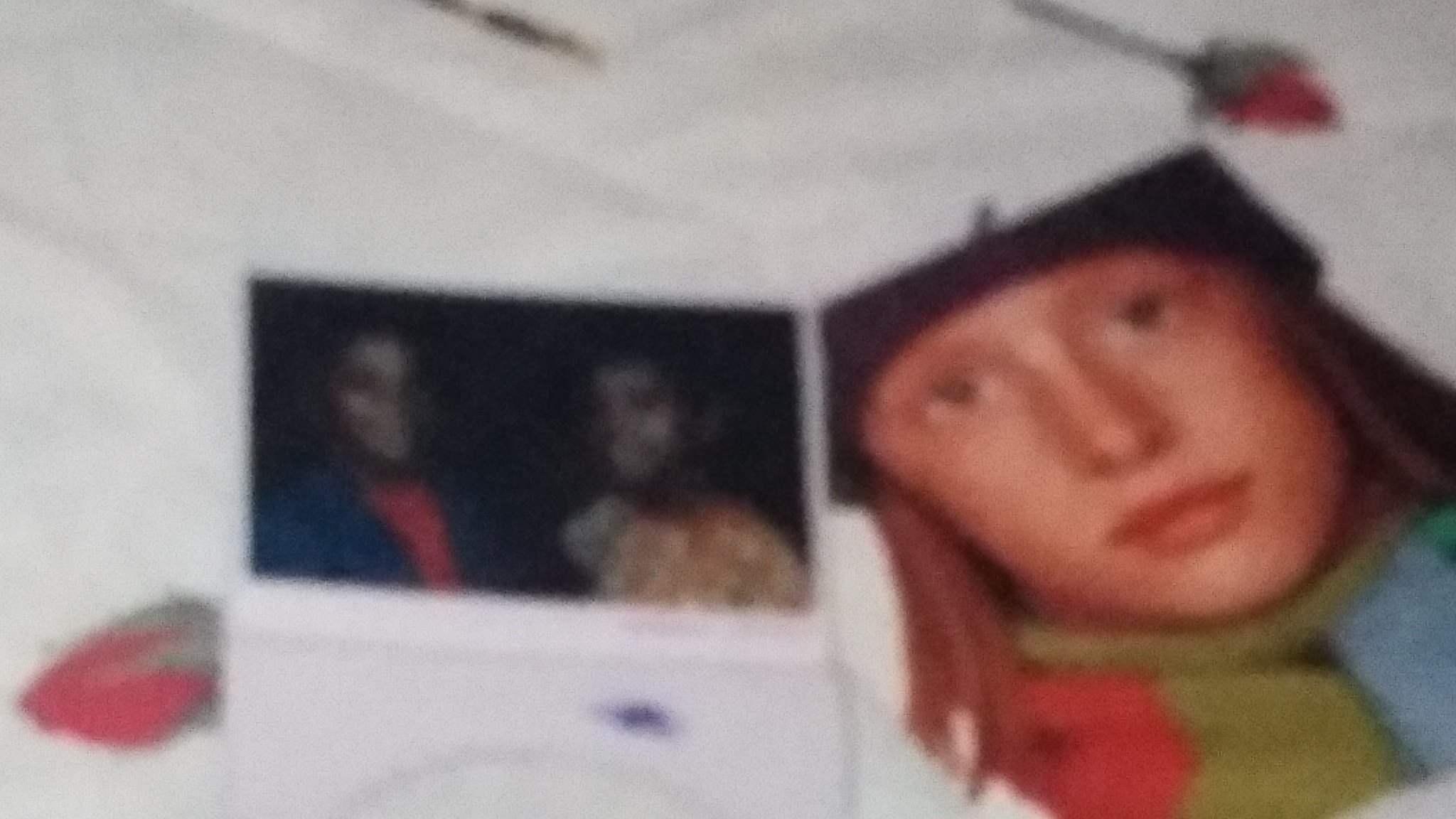In this nostalgic and sentimental scene captured in a very grainy, blurry photo, a collection of photos and mementos are carefully arranged on a tabletop. Most prominently, in the lower right corner, a young woman's face emerges, though her forehead is slightly cut off. Her hair cascades down to her shoulders, and she wears a vividly patterned sweater in hues of blue, green, and red. Just to the left of her image, a photograph of two smiling Black men facing the camera radiates warmth and joy. Beneath their image, a piece of paper lies partially visible, adding a hint of mystery. Adjacent to the paper is a small picture of a vibrant strawberry, its red hue standing out. Completing the tableau, a delicate red rosebud is placed above the young woman's face, adding a touch of elegance and romance to the collection.